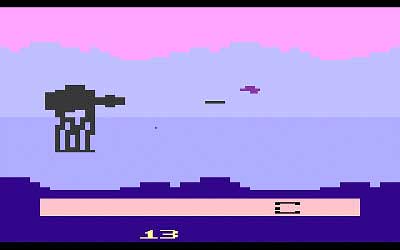This detailed screenshot from the retro Star Wars game on the Atari 2600 depicts an intense battle scene on the snowy planet of Hoth. The backdrop features a gradient sky with a pinkish-purple hue transitioning into light blue, representing the atmospheric layers and ridges of the icy terrain. Central to the image, a black-pixeled AT-AT Walker stands on the left, identifiable by its four legs and distinctive hump. On the right, a purple TIE Fighter approaches, engaged in a daring attack. The game's characteristic Atari-era pixel art vividly captures this iconic Star Wars confrontation. At the bottom, the number "1313" in white letters possibly indicates a scoring or level detail, adding to the nostalgic charm of this vintage game screen.